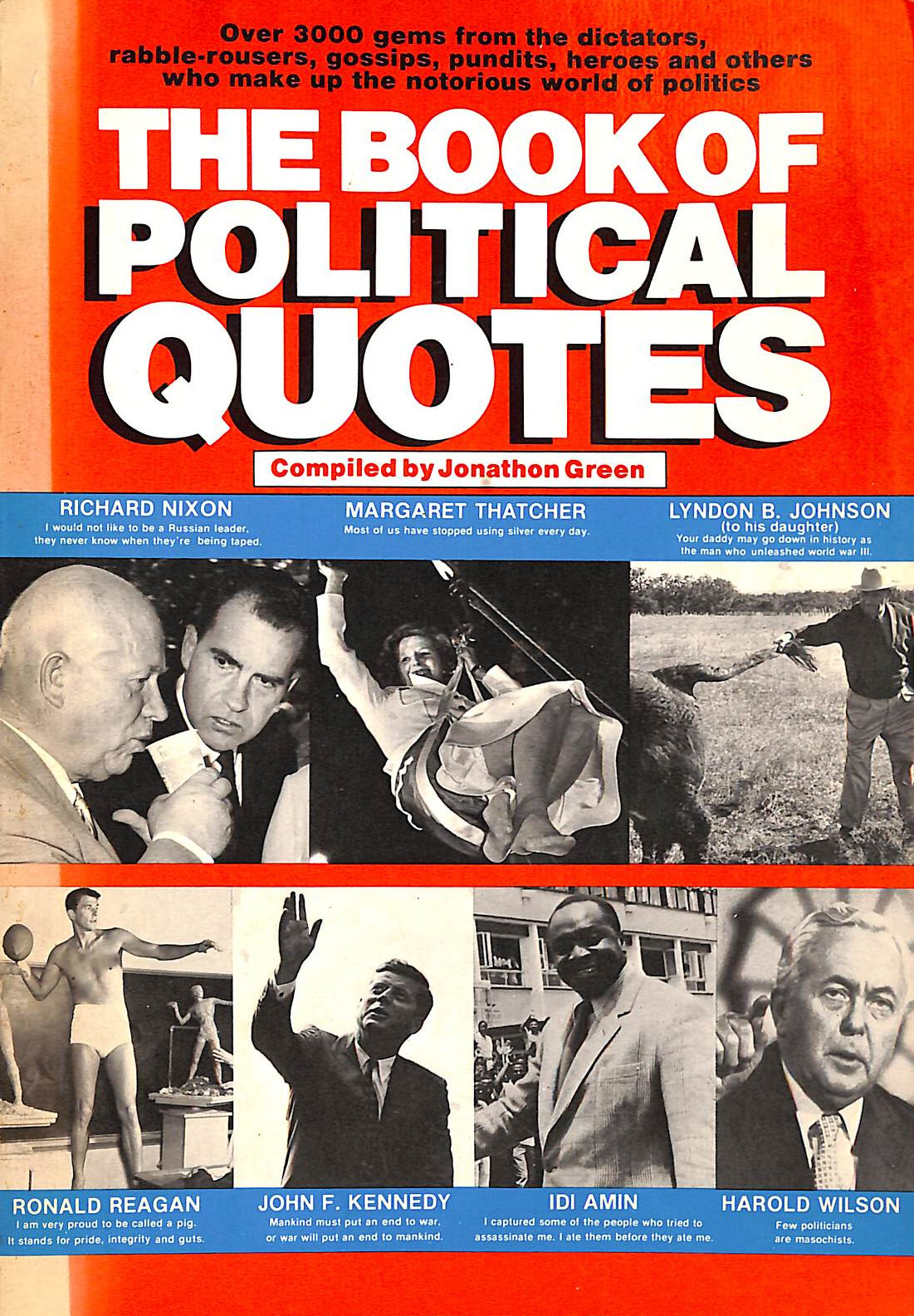This is an image of an orange book cover titled "The Book of Political Quotes," compiled by Jonathan Green. At the top, in black text, it reads, "Over 3,000 gems from the dictators, rabble-rousers, gossips, pundits, heroes, and others who make up the notorious world of politics." Below this, the title "The Book of Political Quotes" is prominently displayed in large white letters. Underneath, in a red font on a white background, are the words "Compiled by Jonathan Green."

The cover features two bands of black-and-white photos, each paired with a notable quote. In the top row, from left to right: Richard Nixon alongside another man with the quote, "I would not like to be a Russian leader. They never know when they’re being taped"; Margaret Thatcher sitting, with the quote, "Most of us have stopped using silver every day"; and Lyndon B. Johnson, depicted hunting and addressing his daughter with the quote, "Your daddy may go down in history as the man who unleashed World War III."

In the bottom row, from left to right: a photograph of Ronald Reagan with the quote, "I am very proud to be called a pig. It stands for pride, integrity, and guts"; John F. Kennedy speaking, accompanied by the quote, "Mankind must put an end to war or war will put an end to mankind"; Idi Amin smiling with the sinister quote, "I captured some of the people who tried to assassinate me. I ate them before they ate me"; and lastly, Harold Wilson with the quote, "Few politicians are masochists." The red background and blue-tinted photo strips create a vivid contrast, making the cover visually striking.